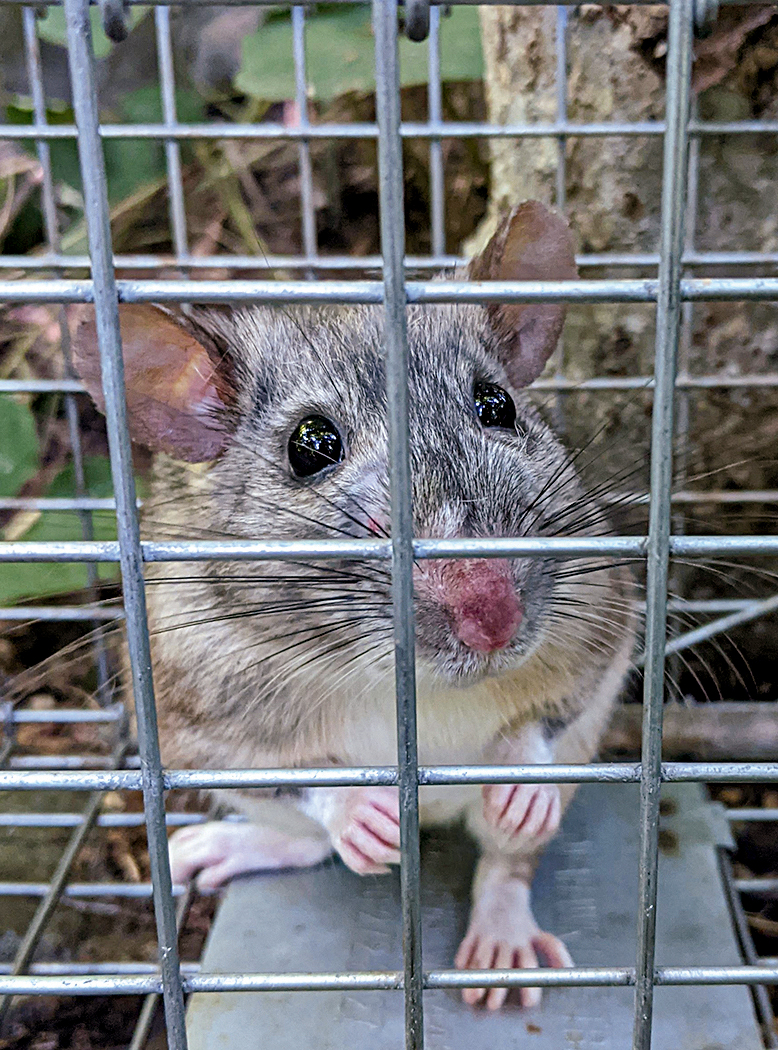The photograph captures a small rodent, likely a mouse, characterized by its glossy, black eyes and mixed fur colors of black, gray, and white. Its large, oval ears, pink on the inside, stand out on its face along with its numerous black whiskers and a pink nose. The mouse stands alert on its hind legs within a grid-like metal cage, which features a square-patterned silver base. The background reveals a natural setting with a leafy green tree, suggesting that the cage might be outdoors. The mouse’s light pink paws are held close to its chest, and it gazes directly at the viewer, seemingly aware of its confinement.